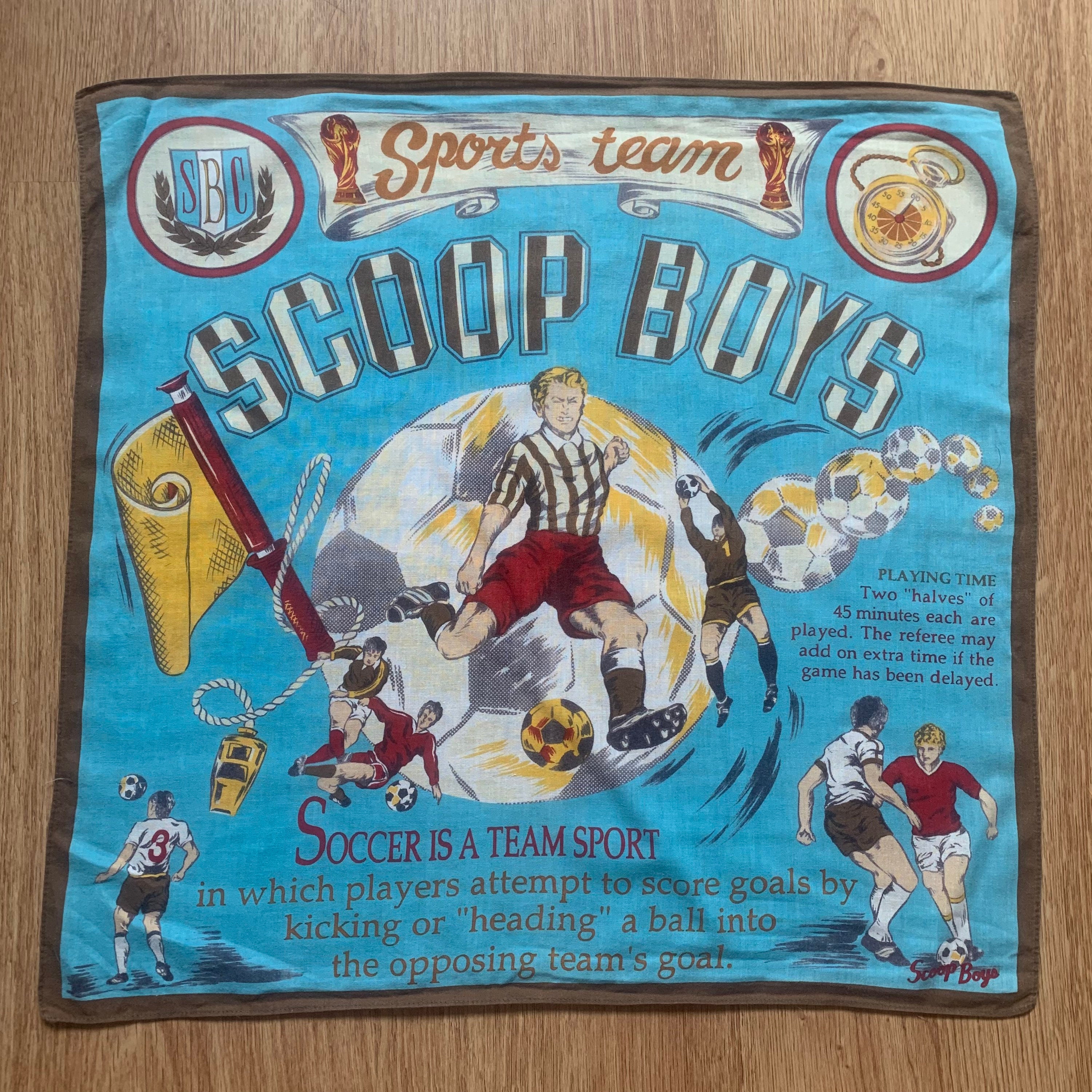This detailed photograph captures a vintage and vibrant handkerchief or printed towel that serves as an advertisement for the Scoop Boys soccer team. The handkerchief features a rich array of soccer-themed imagery and text, set against a color scheme dominated by blue, white, red, and gold, with some brown accents. At the top, a banner reads "Sports Teams," and below is the label "School Boys," alluding to the youthful soccer team it promotes.

Prominently in the center is a circular image of a soccer ball surrounded by various soccer players in action. On the left, a blonde-haired boy or young man, attired in a black and white jersey, red pants, and black socks, is captured mid-kick, striking a yellow and black soccer ball. Adjacent to him, a player dressed in black or brown gear—jersey, shorts, socks, and shoes—is in the action of catching a soccer ball. Lower within the circle, a chaotic moment depicts one player in red falling as he attempts to kick the ball, while another player in black and white is seen leaning over him. 

Surrounding the central image are additional soccer-related graphics, including a flag and a whistle. Also included in the lower sections are detailed textual explanations of the sport: “Soccer is a team sport in which players attempt to score goals by kicking or heading a ball into the opposing team's goal.” Another annotation regarding game rules states, “Playing time: two halves of 45 minutes each are played; the referee may add on extra time if the game has been delayed.”

The handkerchief bears the SBC logo, adorned with laurel leaves, on the left, and a stopwatch graphic encircled in red on the right, further cementing its role in promoting organized soccer play, complete with regulated timing for matches. This artifact not only highlights the excitement and dynamism of soccer but also exudes a charming antiquarian feel, making it a unique collector’s item for soccer enthusiasts.